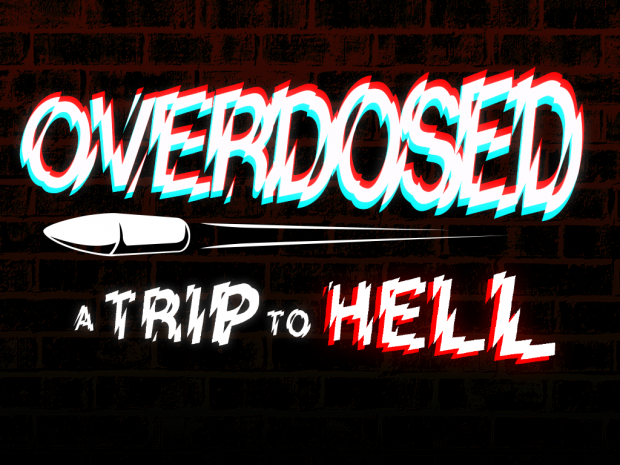The image is a dark, graphic illustration that prominently features the word "OVERDOSED" at the top. This word is rendered in a glitchy, vibrating font with layers of white, light blue, and red, giving it a disorienting, hard-to-focus-on appearance. The background at the top subtly transitions from black to red-outlined bricks, which fade into the dark lower portion of the image. Below the word "OVERDOSED," there is a white bullet streaking towards the left, with lines trailing behind to emphasize its movement. Underneath this bullet, the phrase "A TRIP TO HELL" is written, where "A TRIP TO" is entirely in white, and "HELL" is highlighted in white with a red outline, also appearing to vibrate or shake. The overall composition creates a scattered and unsettling atmosphere, amplified by the chaotic, glitchy text and stark color contrasts.